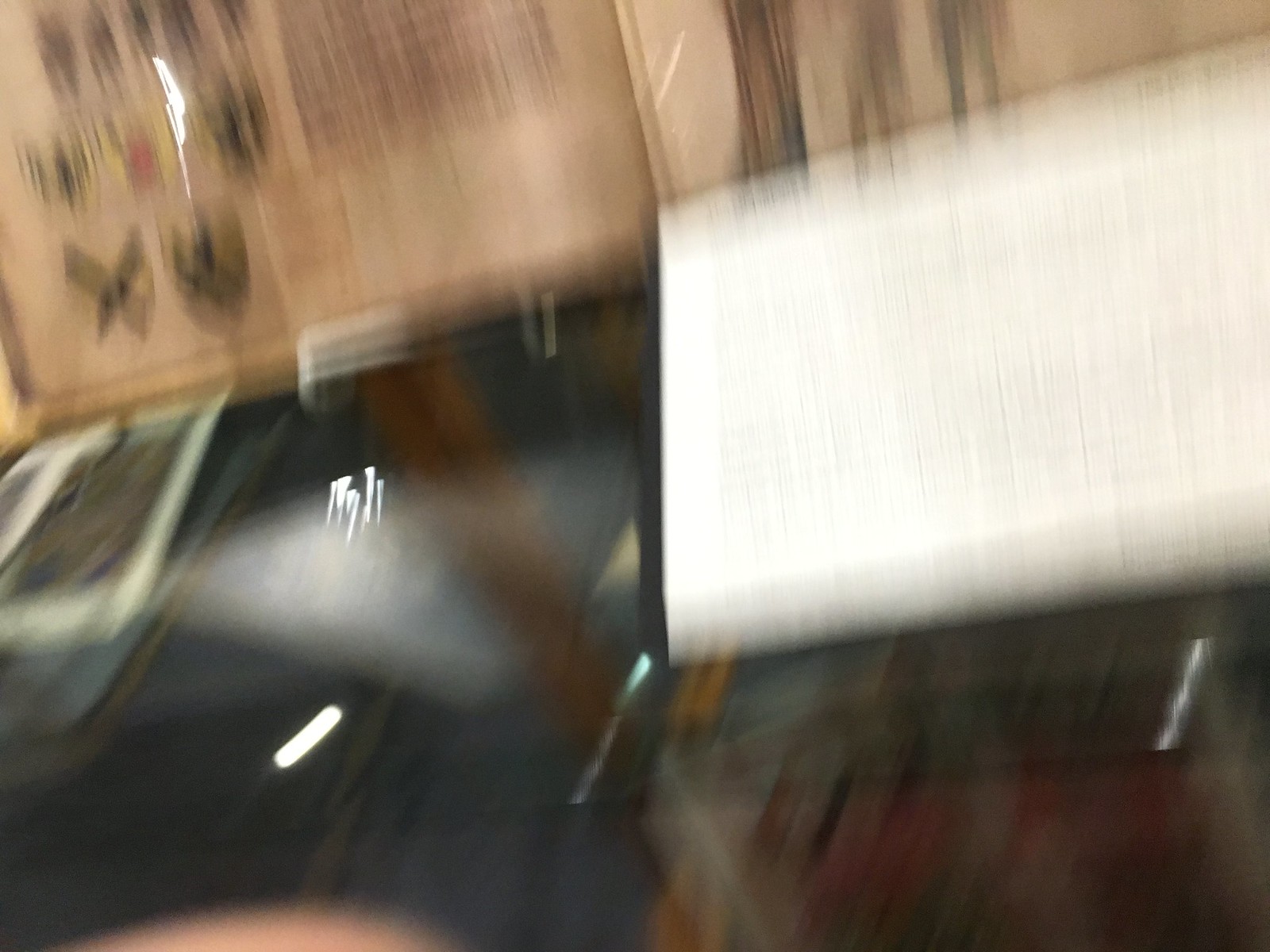A very blurry and out-of-focus photo, making it difficult to discern clear details. In the bottom left corner, there appears to be the top of a hat worn by a person, suggested by the slight curvature of a forehead at the very edge. The top left of the image seems to feature some sort of sign, possibly a billboard. Centrally towards the right, there's a prominent large white sign. The image is interspersed with streaks of light: one in the bottom center, two towards the left of the center, one at the bottom right, and two more at the top, with one on the left and another in the center.